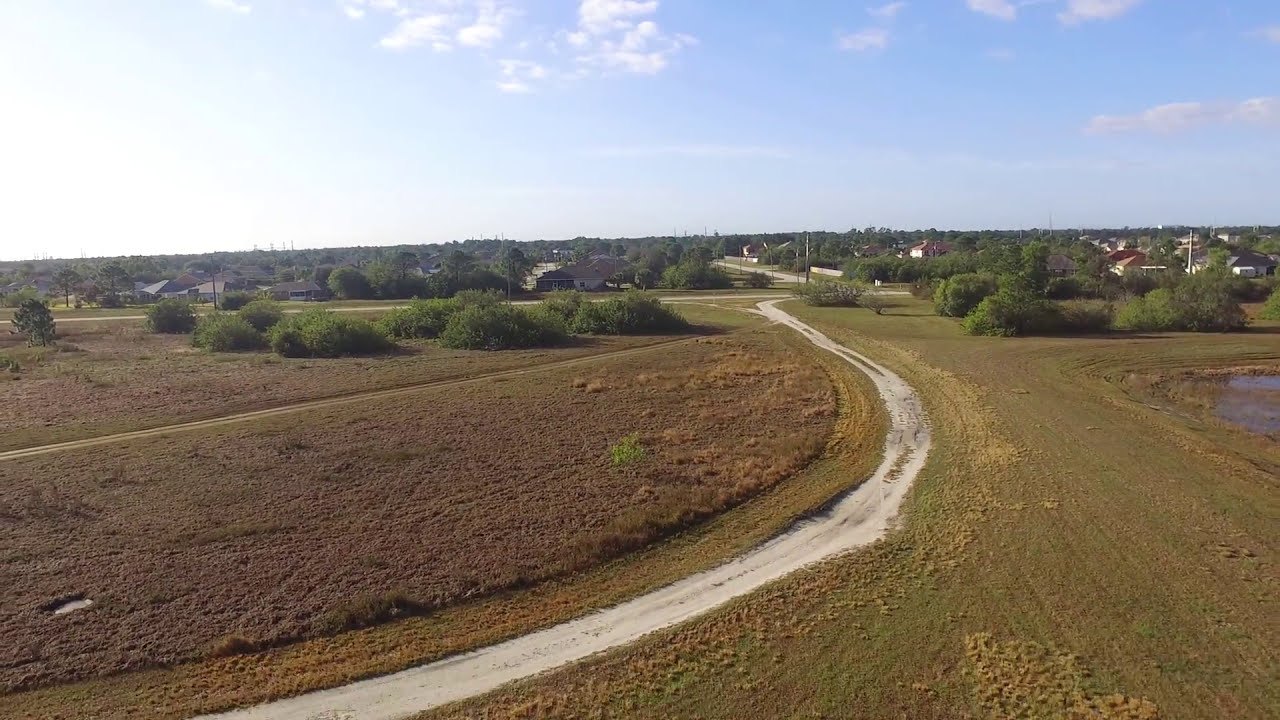The image is a high-angle shot, likely captured by a drone, depicting a serene rural landscape under a clear sunny sky with a few scattered clouds. The focal point is a long dirt road that cuts through a well-maintained grassy area, showing visible lines and patterns, possibly from recent activity or maintenance. To the right of the road is the tip of a pond, surrounded by more grassy fields and small bushy trees. On the left side, there appears to be farmland, with rounded sections possibly growing crops like wheat, crisscrossed by paths that might have been created by ATVs.

As the road extends into the distance, it meets a small two-lane road, bordered by low-lying trees and brush. This road leads into a small rural town with a subdivision of new homes featuring red tile roofs. Power lines run through the neighborhood, and although the town seems distant, it's clear that the area is more developed than the immediate surroundings suggest. The landscape is flat, without any hills or mountains, embodying the quintessential charm of small-town America.